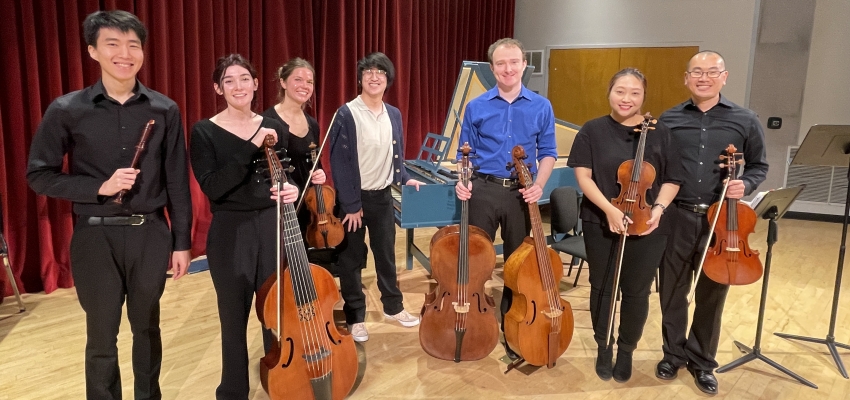In this photograph, a diverse group of seven musicians from an orchestra is posing cheerfully against a red velvet curtain, suggesting they are backstage, possibly during a practice session. They are standing on a light-colored floor, all dressed in black except for a man in a distinct blue dress shirt. The group includes three women and four men, with a mix of Asian and Caucasian individuals.

From left to right, the Asian man on the far left is holding a flute. Next to him stands a Caucasian woman with a large cello. Following her is another Caucasian woman, holding what appears to be either a violin or viola. An Asian man in the middle is seen leaning on a piano, dressed in a white shirt. Next to him, the man in blue is holding two cellos. To his right is an Asian woman with a violin. On the far right, another Asian man holds a violin. Everyone is smiling, enhancing the positive and collaborative atmosphere of the group. The backdrop and the piano hint at a rehearsal space, amplifying the musicians' dedication to their craft.